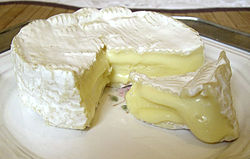This image shows an enticing round dessert, reminiscent of a cake but with several distinct features. The dessert is coated in a smooth, creamy, white frosting that lacks the browned tips typical of a meringue. A triangular slice has been cut out, revealing a vibrant lemon-yellow custard filling that contrasts with the firm exterior of the dessert. The consistency of the custard is clearly evident as it sags slightly from where the slice was removed, creating a sumptuous, rich appearance. The dessert stands two layers tall with frosting not only enveloping the sides but also generously spread on top, making it look extraordinarily appetizing.